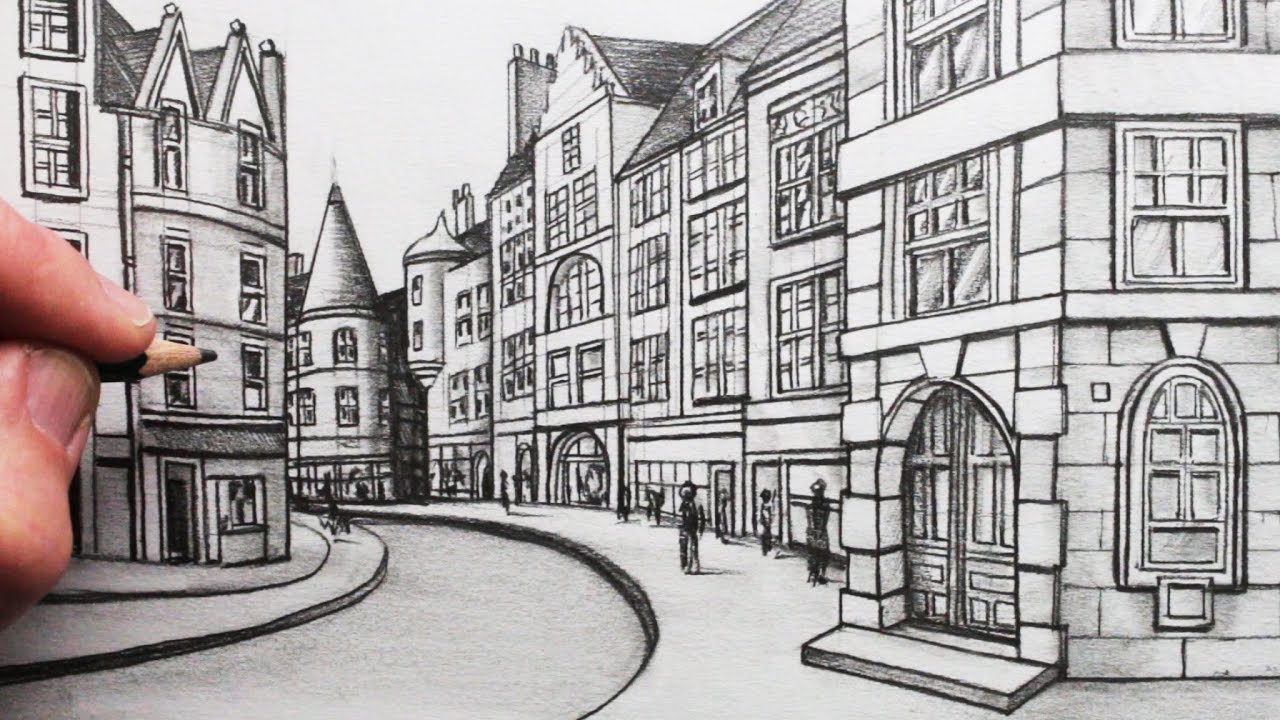This highly detailed, black-and-white pencil illustration depicts a charming medieval European village scene with narrow, winding streets devoid of traffic. The street originates from the bottom left corner of the image, subtly curving up to the right before bending back to the left and disappearing around a corner. The village is characterized by its historic architecture, with squat buildings constructed of bricks and features such as half-crown molding doors and numerous wooden doorways, reminiscent of the 1600s. 

Shadows cast by the buildings create a layered effect, emphasizing the depth and placement of each structure. Sparse clusters of people, drawn as simple silhouettes, populate the sidewalks, contributing to the quaint, everyday atmosphere of the scene. On the left side of the image, a hand holding a pencil intrudes into the frame, showcasing the artist in the process of creating the drawing. The artist's thumb and forefinger grip a black-tipped wooden pencil, poised just above the paper, adding an intriguing meta dimension to the illustration as the creator becomes a visible part of their own artwork.